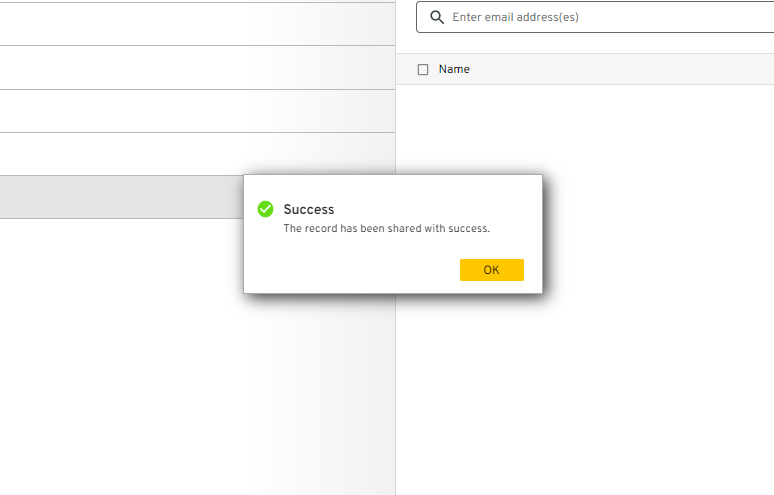The image is a screenshot divided into two distinct sections. On the left-hand side, there is an interface resembling a notepad or notebook with five rows, each separated by four parallel lines. The rows exhibit a gradient starting with an off-white color on the left, transitioning to a darker gray towards the right. The fifth row at the bottom stands out with an even darker gray background, while the upper four rows have a predominantly off-white hue with a light gray tinge moving to the right.

On the right-hand side of the image, there is a search input field with the placeholder text "Enter email addresses." Below this input field, on a light gray background, there is the word "Name" next to an unchecked square checkbox. Centrally located is a rectangular notification box, slightly shaded for emphasis, displaying the word "Success" accompanied by a green checkmark. Beneath the success message, it reads, "The record has been shared successfully." At the bottom right of this notification box is a yellow "OK" button.